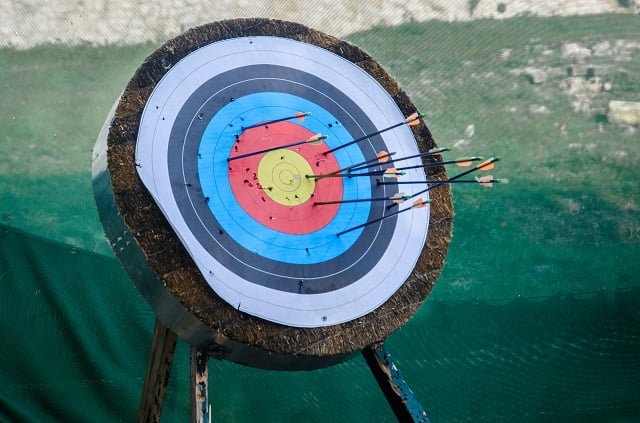This photograph captures a detailed, horizontally aligned close-up of an outdoor dartboard scene. The blurred background features a blend of green grass and scattered white and light gray rocks, possibly indicating the edge of a retaining wall in the upper portion from left to right. The central focus is a round piece of wood, reminiscent of a tree stump, resting on three visible narrow, rectangular wooden legs with chipped paint.

Mounted on this wooden base, there's a circular, paper target comprised of ten concentric rings transitioning in color from the outermost circles of white, to dark blue, light blue, red, and culminating in a yellow bullseye at the center. The target has several darts lodged in it, notably avoiding the white rings. Instead, the darts are dispersed across the dark blue, light blue, red, and one marks the yellow bullseye area. The overall scene suggests a well-used target setup amidst a natural, green, and rocky backdrop.